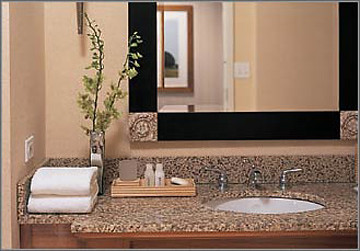This detailed color photograph showcases a portion of a serene bathroom interior. Central to the image is a pristine white sink adorned with sleek silver fixtures, including the faucet and hot and cold nozzles. The countertop surrounding the sink is an exquisite dusty rose granite, interspersed with flecks of gray and black, providing a touch of elegance.

On the far left side of the counter, a neatly stacked pair of white towels adds to the bathroom's clean and inviting look. Adorning the counter is a tall, slender silver vase holding two delicate branches with white flowers, injecting a hint of natural beauty into the space.

The walls are painted a subtle, light pink hue, enhancing the room's soft and calming atmosphere. Above the sink hangs a mirror, which reflects the opposite wall, continuing the pink color scheme. The reflection also reveals a couple of framed photographs or posters, adding a personal and artistic touch to the decor.

Also situated on the counter is a small wooden tray. This tray holds a bar of white soap, two small plastic bottles, and a small gold-toned object towards the left, further completing the picture of refined simplicity and comfort in this bathroom space.